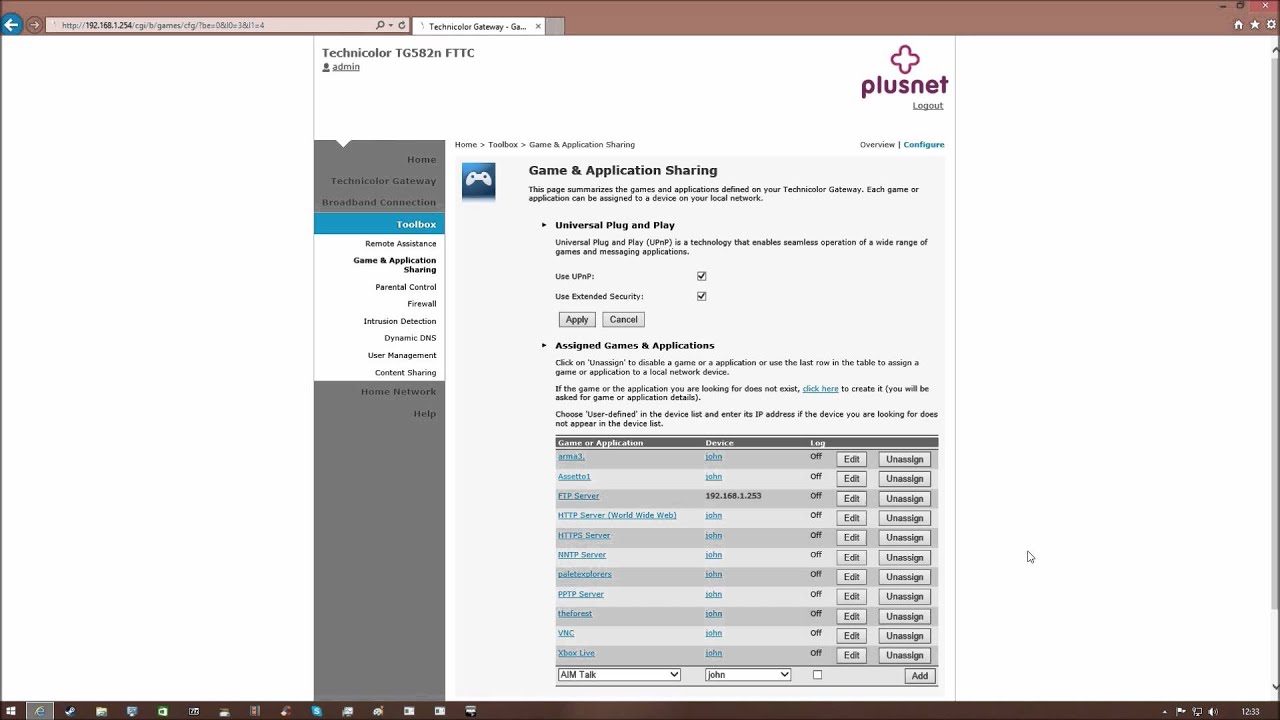This image is a detailed screenshot of the Plusnet web page, specifically illustrating the Technicolor TG582n FTTC demonstration interface. 

At the top of the screen, there's a brown navigation bar featuring various symbols on the far right and a search bar on the left. Centered in the upper right corner is the Plusnet logo in blue or purple, characterized by a plus sign above it. Next to the logo, there's a "Logout" option.

The page layout is divided into two columns. The narrow column on the left has a gray background and features several navigation options. It includes a blue bar labeled "Toolbox," below which options like "Remote Assistance," "Games and Application Sharing" (highlighted in bold), "Parental Control," "Firewall," "Intrusion Detection," "Dynamic DNS," "User Management," and "Content Sharing" are listed. Further down, it shows links to "Home Network" and "Help" sections. Above, quick links to "Home," "Technicolor Gateway," and "Broadband Connection" are displayed.

The right side of the page is a much broader column focusing on "Games and Application Sharing." This section begins with a title bar stating "Home > Toolbox > Game and Application Sharing." Below this, a blue-highlighted box explains "Universal Plug and Play" (UPnP) technology, which supports the seamless operation of various games and messaging applications. The section ticks off UPnP’s features such as user extensibility and extensive security, with checkmarks indicating enabled settings. There are "Apply" and "Cancel" buttons beneath these settings.

Further down, the interface allows for the assignment and management of games and applications. This section offers a table with gray headings for "Game or Application," "Device," and "Logged On/Off." Users can manage each game or application with "Edit" and "Unassign" buttons. This functionality enables users to assign specific games or applications to particular local network devices, effectively managing network resources devoted to gaming.